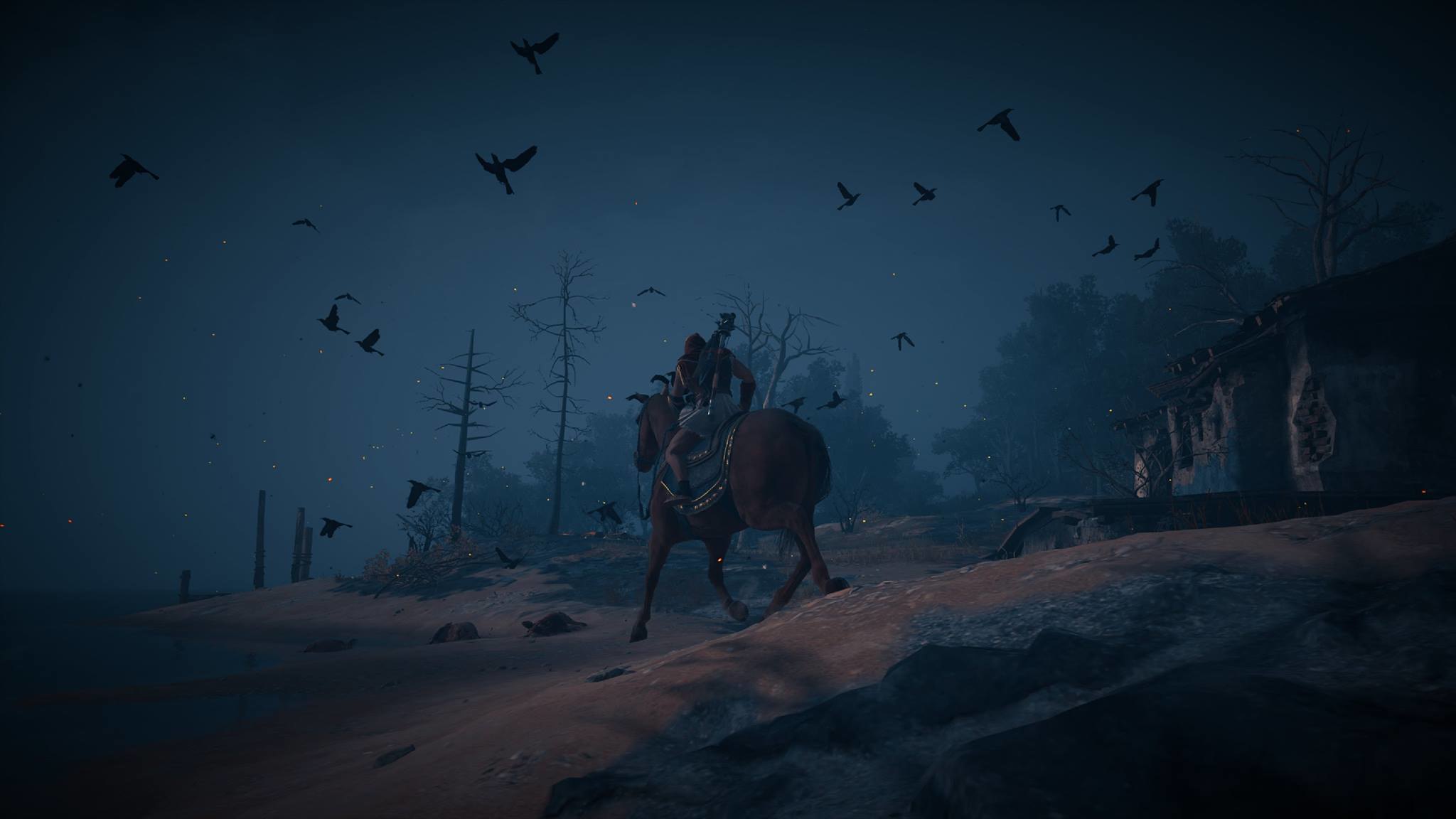The digital art piece depicts a nighttime scene, heavily shadowed and imbued with a sense of mystery. Central to the image is a brown horse, viewed from behind as it travels away from the viewer towards a darkened tree line. The elaborate saddle it bears is adorned with a gold-rimmed blue blanket, highlighting its ornate craftsmanship. Atop the horse sits a rider, mostly indistinct in the heavy shadows but seeming to carry something possibly weapon-like strapped to their back, and their left leg is secured in a visible stirrup.

In the dark blue night sky, dotted with bright yellow stars, a swarm of black birds—likely crows—circles around the rider in various stages of flight, adding to the ominous atmosphere. The landscape they traverse appears barren, with patches of dead grass or driftwood underfoot and skeletal trees devoid of leaves. To the right of this central scene stands a dilapidated structure, possibly a hut or building with a log roof, constructed from stone. The mix of bare-branched trees and those with dense, possibly evergreen foliage, casts eerie silhouettes against the horizon, contributing further to the scene's haunting aura.